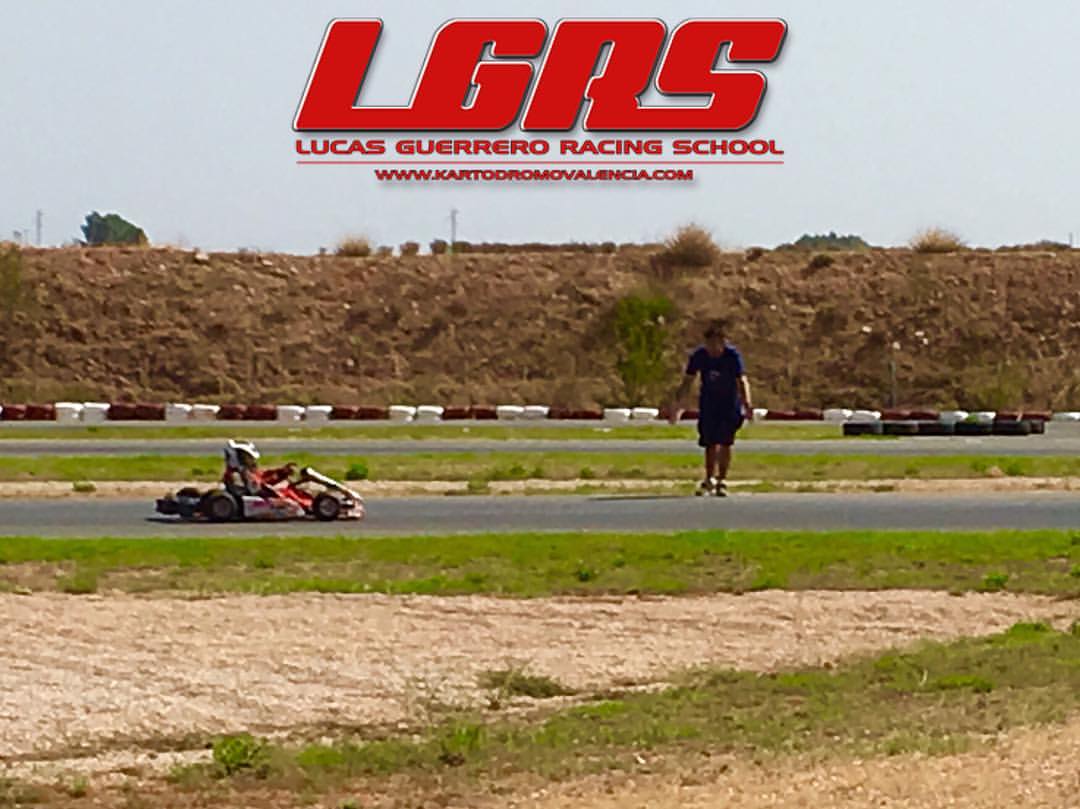The image is a vibrant, full-color advertisement for the Lucas Guerrero Racing School (LGRS). The sky has a gray haze, suggesting a cloudy day. Prominently displayed in red font at the top are the words "Lucas Guerrero Racing School," accompanied by the initials "LGRS" in large block letters, and the website "www.kartodromovalencia.com" embossed over the sky. The scene shows a go-kart track with a person, likely a child, driving a red and white go-kart while wearing a helmet. A man dressed in a dark t-shirt and black shorts stands nearby, possibly an instructor, observing or giving directions. The track is surrounded by a mix of grassy patches, some brown, and sandy areas, with tires lining the track to prevent the kart from veering off. In the background, a mound of dirt and a small hill with a few trees and wooden poles add to the detailed landscape of this go-karting environment.